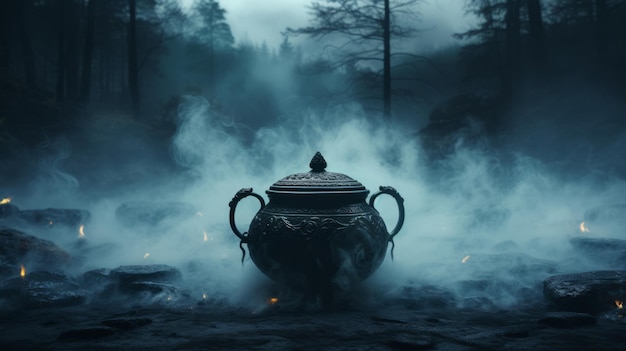The image, an artistic photograph or a movie screenshot, presents a central bulbous vase with two semi-circular handles on either side, and a small conical handle on its lid, which can be lifted. Surrounding the vase are smooth, black, flat rocks and small lit candles, producing an eerie smoke that envelops the area. Tiny sparks or flames flicker amidst the smoke. In the dark, sinister background, various bare trees and dark-colored vegetation are visible under a gloomy, dark gray sky. The overall color scheme is dominated by shades of black, white, dark blue, and the orange hues of the flames. The ominous atmosphere suggests something malevolent about the vase.